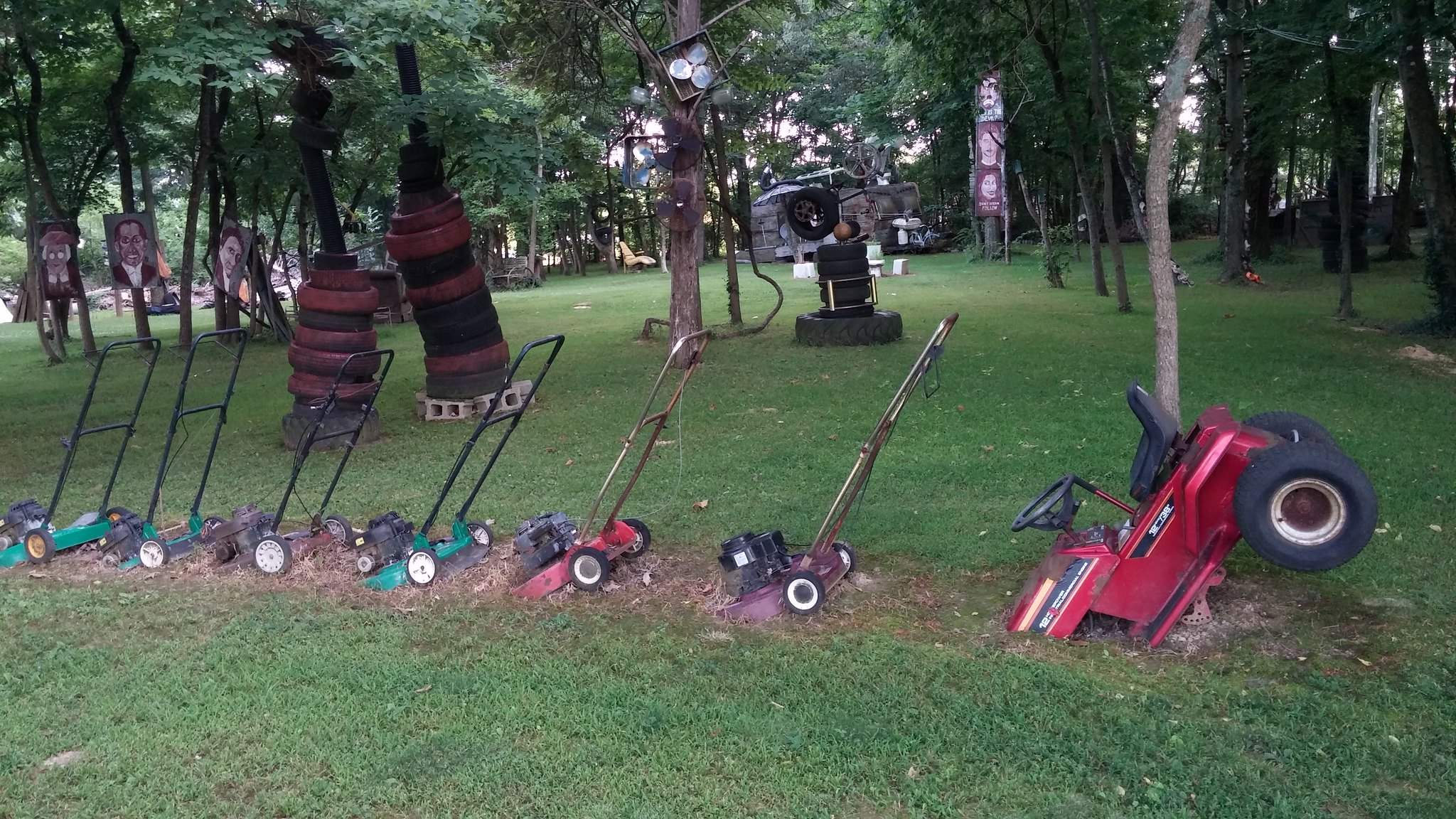In a verdant, flat park enveloped by trees, stands a captivating art installation merging whimsical and rustic elements. Dominating the foreground is a row of lawnmowers—green, red, green, red—buried diagonally into the earth, leading to a partially buried ride-on tractor. Adjacent to this intriguing lineup, a red toy car is similarly embedded, with only its back wheels and seat exposed. Behind this, an eclectic collection of sculptures emerges: a stack of tires mounted on a pole with cinder blocks at its base, another tire paired with a tree adorned with wind chimes and fans attached to its trunk. Adding to the gallery are totem pole-like structures scattered throughout. On the left side, three portraits dangle from trees, their somber faces framed by the lush foliage. A variety of other artworks, including metal sculptures and paintings, embellish the scene, while hints of a camper or rustic structure peek from the background, enhancing the sense of an outdoor haven devoted to imaginative reuse of everyday objects.